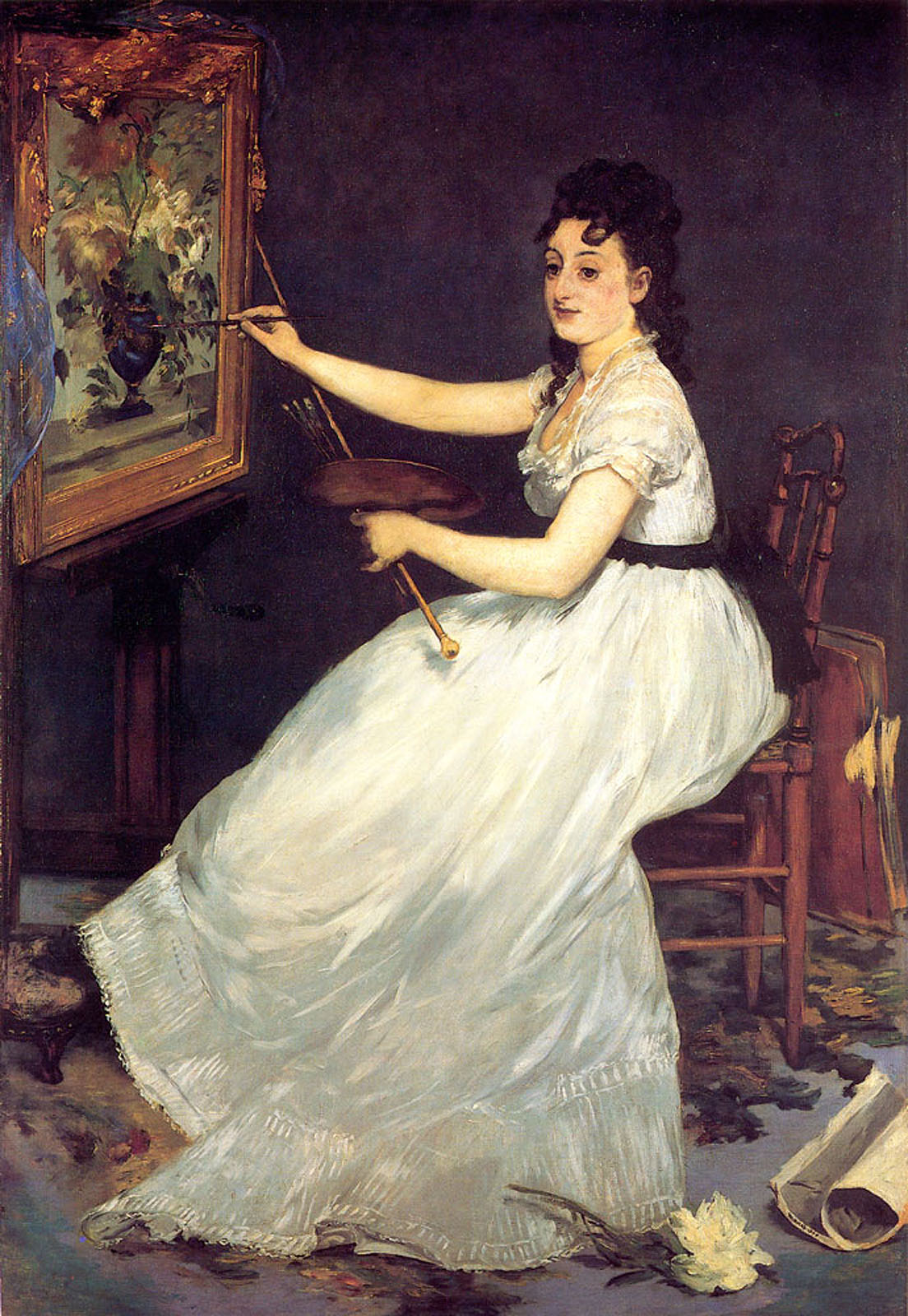The image is a detailed painting depicting a woman with long black curly hair sitting in a wooden chair, centrally positioned. She is wearing a long, elegant white gown with a black waistband, resembling a wedding dress. In her left hand, she holds an artist's palette, while her right hand wields a paintbrush. The woman is engaged in painting a flower vase set in a richly adorned frame with golden borders and intricate designs, located at the top left of the image. 

The background of the room is a deep, dark purple, adding a regal ambiance to the scene. Scattered on the floor around her are various items, including papers, a large flower, and what appears to be dirt and debris, giving a somewhat cluttered yet natural look. Beneath the chair, a carpet can be seen, and behind the chair, there are additional papers or possibly a book. The overall composition, colors, and elements evoke a sense of refinement and artistry, akin to a scene one might expect to find in a museum piece.